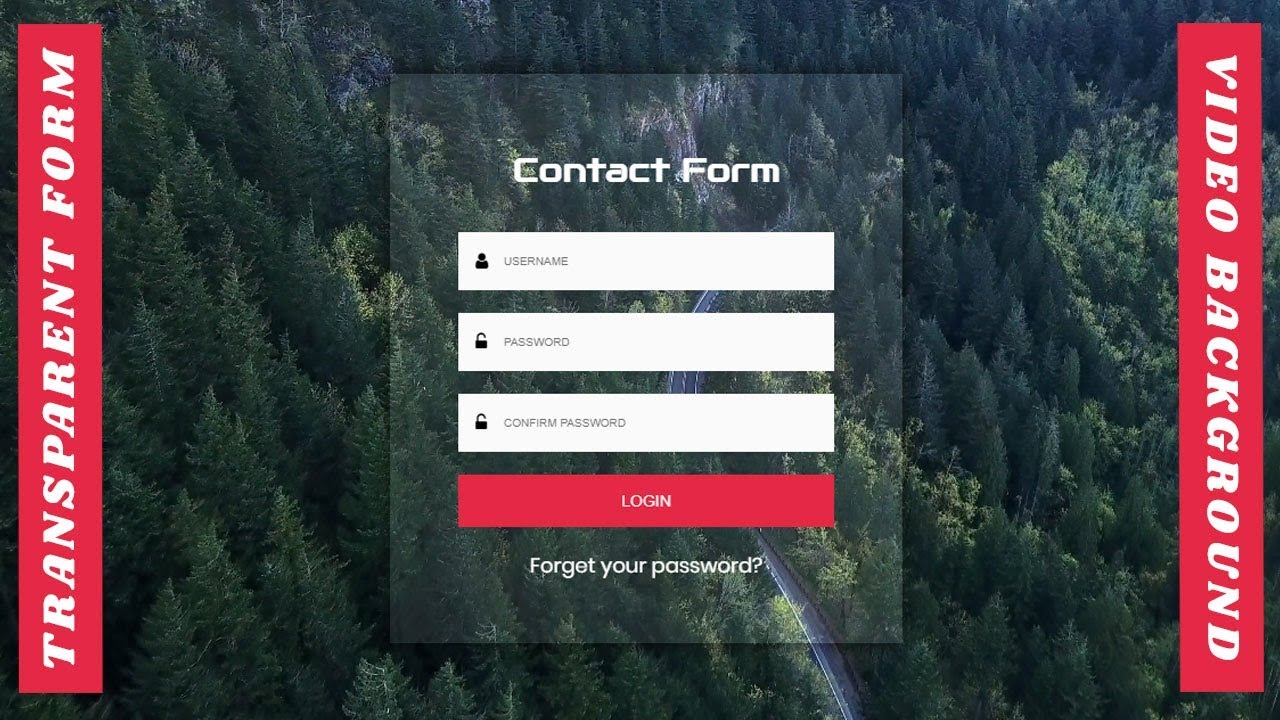Screenshot of a website showcasing a scenic pine forest landscape. The image depicts a winding road that begins at the bottom center of the screen and curves its way up towards the right, set against a backdrop of lush pine trees climbing a mountain slope towards the upper left. Overlaying this picturesque background, there are two red banners with bold white block text: "Transparent Form" on the left side, starting from the bottom, and "Video Background" on the right side. 

Centrally positioned on the image is a "Contact Form" featuring the following elements:
- A white input box labeled "User Name" with a small person icon.
- Below it, an input box for "Password" accompanied by a lock icon.
- Another input box for "Confirm Password," also indicated with a lock icon.
- Finally, a red action button labeled "Login" at the bottom.